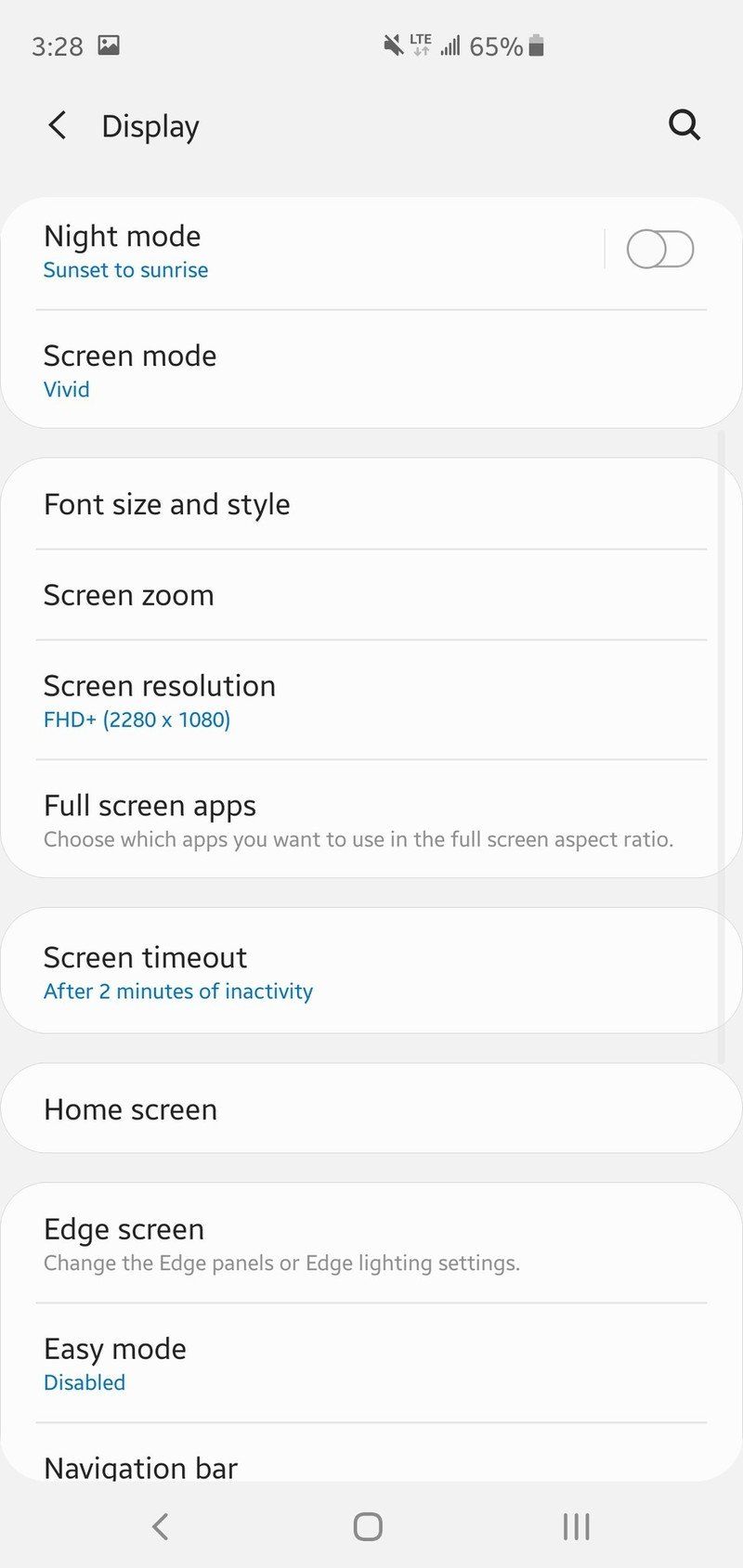The image displays an interface with a light gray background, transitioning to a white background on the top left, marked "328". To the right of "328" is a small, square image icon. Adjacent to this, on the left, is a gray arrowhead pointing left with the word "Display" next to it. On the far right is a gray magnifying glass icon.

Centered in the interface is a white rectangular area with rounded corners. It features the words "Night mode" in black text, and below it in small blue text, "Sunset to sunrise." There is a toggle switch to the right of this text, currently turned off. Beneath this section is a light gray divider. The subsequent section, labeled "Screen mode," has black text and "vivid" written in small blue lettering underneath.

The gray background reappears, leading into another larger white rectangular area with rounded corners. The top of this section, marked "Font size and style" in black text, is followed by a divider line, then "Screen zoom" in black text. Another divider separates this from "Screen resolution" in black, with "FHD+" and "2280 x 1080" in blue text beneath. Following another gray line divider, the text "Full screen apps" appears in black, with a smaller gray font explaining, "Choose which apps you want to use in the full screen aspect ratio."

The interface transitions back to the light gray background, featuring another white rectangular section with rounded corners. This section is labeled "Screen timeout" in black text, stating "After two minutes of inactivity" in small blue letters underneath. Further down is another white, slightly more oval-shaped area labeled "Home screen" in black text.